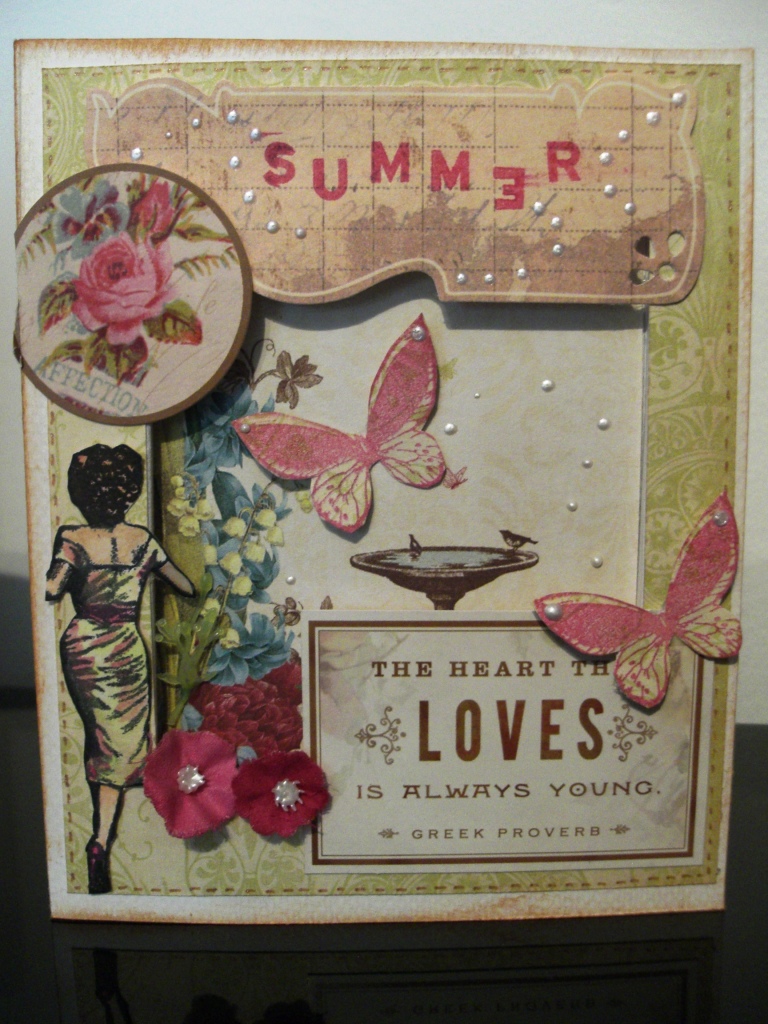The image depicts a detailed and textured art project, possibly a greeting card or scrapbook page, propped upright on a shelf with a supportive backing. The centerpiece features a vibrant 3D collage combining various decorative elements. At the top, the word "summer" is prominently displayed in red letters, with a distinctively backward "E" that gives it a handmade charm. Scattered across the piece are intricately attached butterflies, enhancing the three-dimensional effect. 

In the bottom left corner, there's an illustration of a woman in a dress, running away from the viewer, amidst textured poppies. The center is graced by a combination of blue and white fabric flowers with a birdbath illustration adding to the scene. Additional butterfly decorations, along with real flower embellishments, further enrich the visual appeal. Small silver dots, resembling pearl embellishments, are dispersed throughout, adding a touch of sparkle.

Towards the bottom right, a quote reads “The heart that loves is always young,” attributed to a Greek proverb. Behind one butterfly, part of the text may be obscured, adding an element of curiosity. This lovingly adorned piece, replete with flowers, butterflies, and thoughtful quotes, reflects a meticulous and creative hand, making it more than just a simple art project.